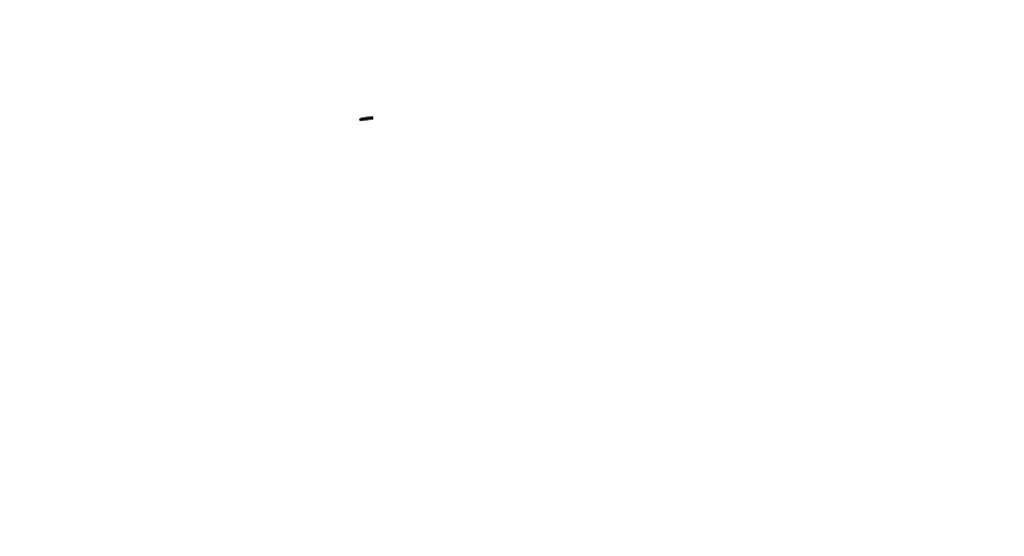The image depicts an almost entirely blank white background with two small, indistinct marks. On the left side, there is a small dark grey mark that appears to be either a dash or three closely clustered circles, although the precise shape is indeterminate. To the right of this dark grey mark, barely visible, is an even fainter light grey mark. This light grey mark, approximately half the size of the dark grey one, also seems to be either a dash or a few closely packed circles. The dark grey mark is somewhat nondescript and not particularly dark, while the light grey mark is extremely pale, making it difficult to discern its exact form.